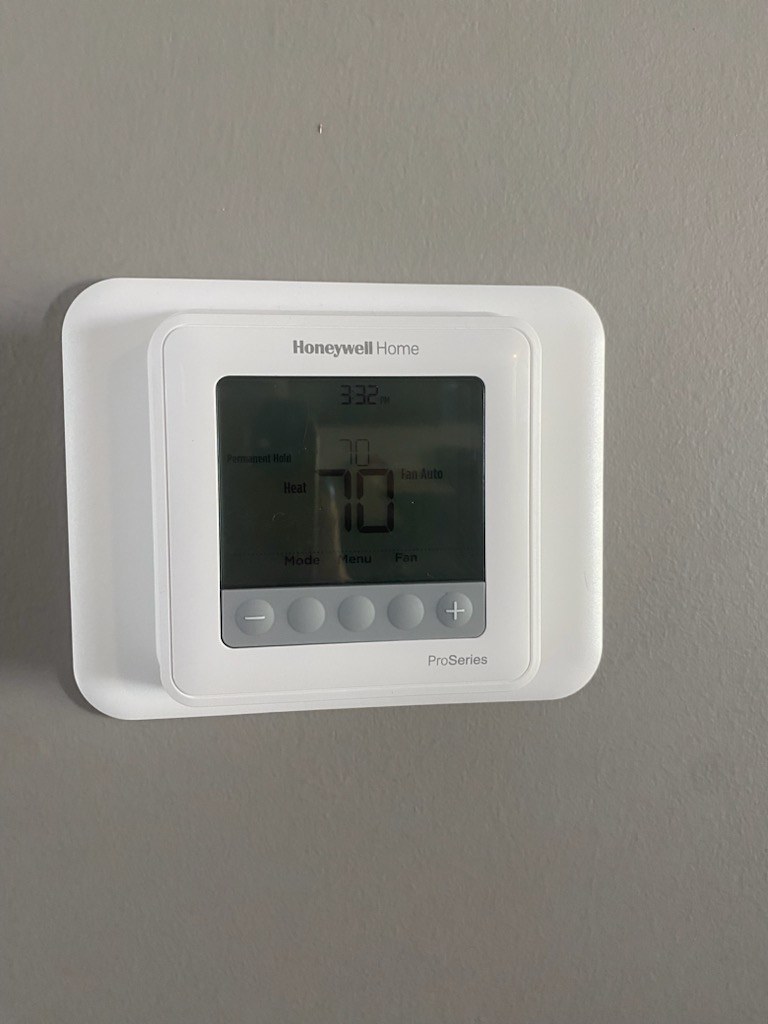This image features a Honeywell Home Pro Series programmable thermostat mounted on a light gray wall. The thermostat itself is predominantly white with a sleek plastic face. The device includes a white base and a raised control area that features five gray buttons, positioned horizontally from left to right. The buttons are labeled with negative and positive symbols on either end for easy adjustment. The thermostat's display shows the current time, 3:32 p.m., and indicates that the temperature is set to 70 degrees Fahrenheit, which matches the current ambient temperature. Additional display information includes the status indicators for 'Heat', 'Mode', and 'Alarm'. The fan setting is on 'Auto', ensuring optimal climate control. The bottom of the thermostat bears the inscription 'Pro Series' just below the buttons, indicating its model.